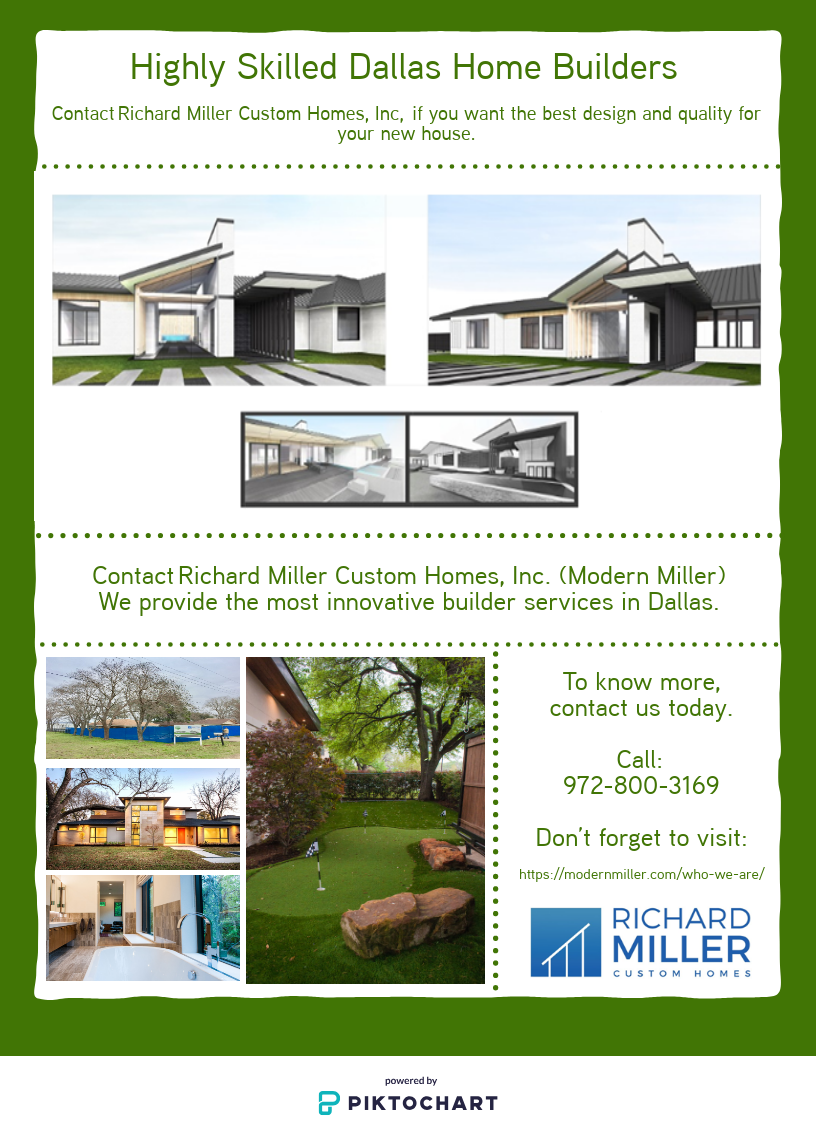The image is a detailed brochure with a white background and a green border, primarily text-based with several images. At the top center in green text, it reads "Highly Skilled Dallas Home Builders." Below, in smaller green text, it encourages potential clients to "Contact Richard Miller Custom Homes Inc. if you want the best design and quality for your new house." The brochure features four images showcasing modern, single-story homes with white exteriors and black roofs, including two larger images and two smaller ones. 

In the center of the brochure, it states, "Contact Richard Miller Custom Homes Inc. (Modern Miller). We provide the most innovative builder services in Dallas." Toward the bottom left, there are additional images: a sizable one depicting a home's backyard with a putt-putt course, artificial rocks, and bushes, alongside three smaller images of home exteriors and interiors.

At the bottom right, in green text, it reads, "To know more, contact us today. Call 972-800-3169. Don't forget to visit," followed by a website URL, "modernmiller.com," though the text is too small to read clearly. The logo featuring "Richard Miller" in blue with "Custom Homes" in smaller text below is accompanied by a blue square with a white 2D rooftop image. The brochure concludes with "Powered by Piktochart" in black text at the very bottom.